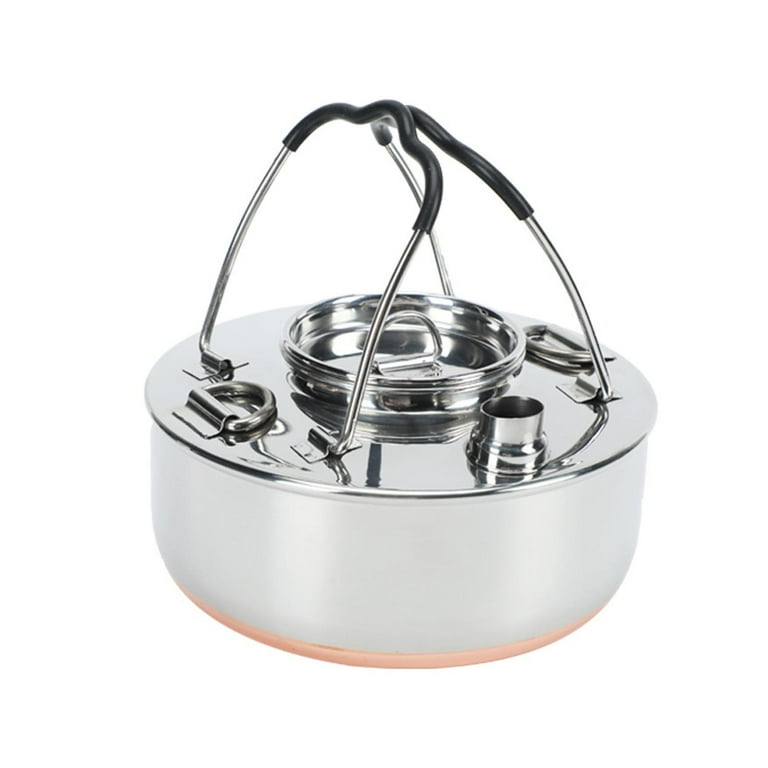This image is a close-up of a metal pot with intricate details. The background is entirely white, isolating the pot as the sole focus. The pot features two thin metal handles with black rubber grips at the top, designed for easy and safe handling to prevent burns. These handles can fold up and down and meet at the top, reminiscent of the shape of a stethoscope.

The lid of the pot is primarily silver, adorned with several silver latches and a circular twist handle in the center, which acts as a screw-open mechanism. There's a small circular opening on the lid, seemingly intended for pouring liquids or adding contents. Just beneath the lid, the body of the pot is white, seamlessly transitioning into a copper or light orange color at the base, adding a touch of warmth to its appearance.

The pot lacks any branding or writing, maintaining a minimalist aesthetic. Its overall design suggests functionality, possibly serving as a specialized container for liquids, resembling a tea kettle with its practical features and visual appeal.